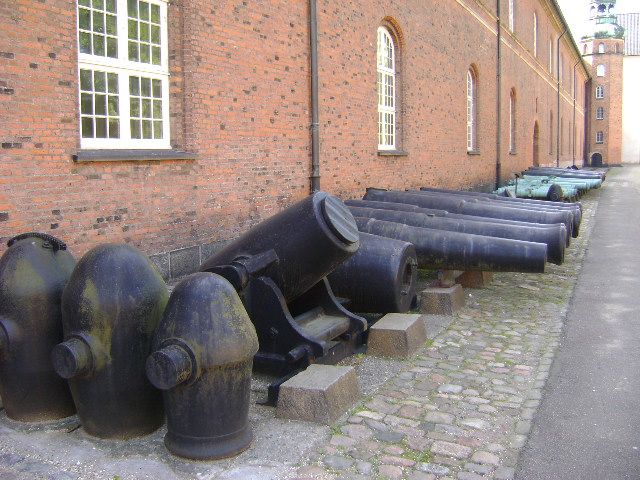The image captures an outdoor scene along a brick building as viewed from a sidewalk. In the foreground, a series of very old cannons are lined up, all pointing to the right. There are two short, stubby cannons and several longer, thinner ones, some of which overlap each other making it difficult to count, but it appears to be about six or seven black cannons and at least two light blue ones. Some cannons have plugs with rocker arms, and there's a barrel positioned upright with a plug in it. Heavy iron anvils and cylinders are scattered around, likely related to the cannons. The brick building occupies the top two-thirds of the image with a series of windows and poles running vertically. It features a window with white trim and multiple panes of glass, followed by more windows interspersed with metal poles, and culminating in a large, five-story tower with a column of windows above a distant door. In front of the cannons, a brick walkway extends along the side of the building, transitioning into cobblestones that lead to a paved road on the right.